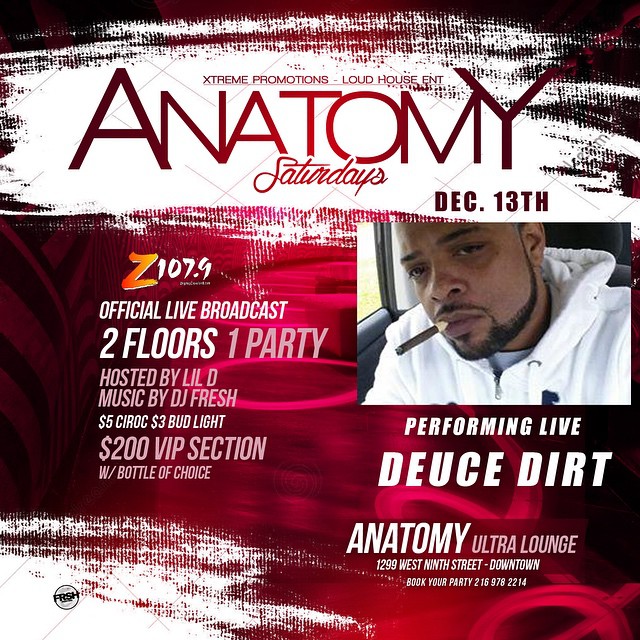The promotional poster for Anatomy Ultra Lounge is a vibrant and dynamic piece of graphic design, blending illustration and photographic elements. The square format features a dramatic red background with a darker red, tornado-like spiral at the center, creating a sense of motion and intensity. At the top, a broad white streak stretches horizontally, adorned with the bold, dark red text "Extreme Promotions Loud House ENT" followed by the headline "ANATOMY SATURDAYS" in a script font, alongside the date "December 13th" on the lower right of this section.

Beneath this heading, there is a square photograph of an African-American man wearing a white hooded sweatshirt, seated inside a vehicle, smoking a cigar and gazing downward. To the right of the photograph, white block lettering announces "Performing Live Deuce Dirt."

The left side of the poster provides event details, starting with the sponsor logo "Z107.9 Official Live Broadcast." Below, in white and light pink text, are the specifics: "Two floors, one party hosted by Lil D, music by DJ Fresh," alongside drink specials "$5 Ciroc and $3 Bud Light" and a VIP offer "$200 VIP section with Bottle of Choice." 

In the poster’s bottom right corner, additional details for Anatomy Ultra Lounge's address are provided: "1299 West 9th Street Downtown. Book Your Party 216-978-2214." The lower left corner features another streak of white, possibly containing a small black circular logo.

The combination of blurred red backgrounds, bold typography, and striking imagery creates a compelling and energetic advertisement, effectively capturing the essence of the event and its exclusive offers.